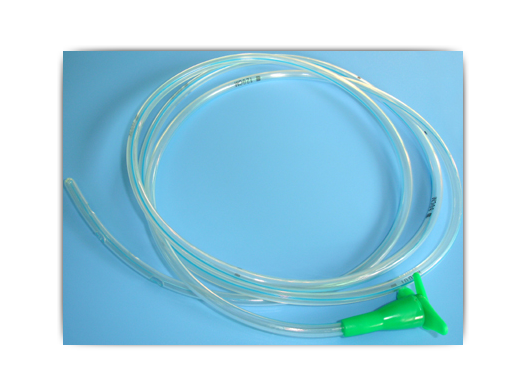The image features a long, clear plastic tube set against a light blue background. The tube, resembling a thick straw, is coiled in large, circular loops—three or four times—occupying most of the frame. The opening of the tube is located at the left middle edge of the image, while the coils extend across the picture, with some loops touching the right edge and the top middle of the frame. A distinctive feature is a bright green, V-shaped attachment at the tube's end, situated near the bottom of the image. Periodically along the tube, there are small black text markings, presumably product numbers, though they are too small to decipher. The upper left corner of the background shows some darker shadowing, adding depth to the scene.